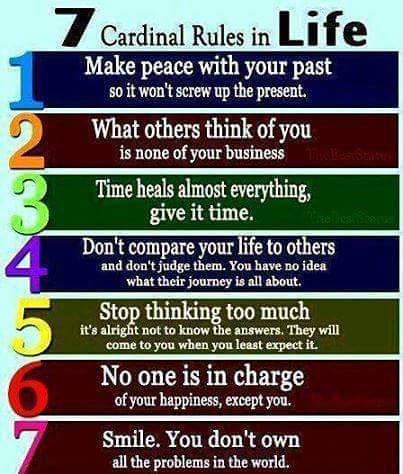The image showcases a motivational poster entitled "Seven Cardinal Rules in Life" displayed on a light blue background. The heading is written in bold black font. The list consists of seven horizontally aligned, rectangular bars, each distinctively colored and numbered. Each rule is written in white font against a colored box. The detailed breakdown of the rules, with corresponding colors, is as follows:

1. A dark blue bar with the text: "Make peace with your past so it won't screw up the present."
2. An orange box with the inscription: "What others think of you is none of your business."
3. A dark green bar that reads: "Time heals almost everything, give it time."
4. A dark purple box containing the words: "Don't compare your life to others and don't judge them. You have no idea what their journey is all about."
5. A greenish-yellow bar with the message: "Stop thinking too much. It's all right not to know the answers. They will come to you when you least expect it."
6. A dark red box that states: "No one is in charge of your happiness except you."
7. A dark pink bar with the final rule: "Smile. You don't own all the problems in the world."

The colorful presentation and varied shades underscore the motivational message, making it visually engaging and uplifting, akin to a slide you might see in an inspirational presentation.